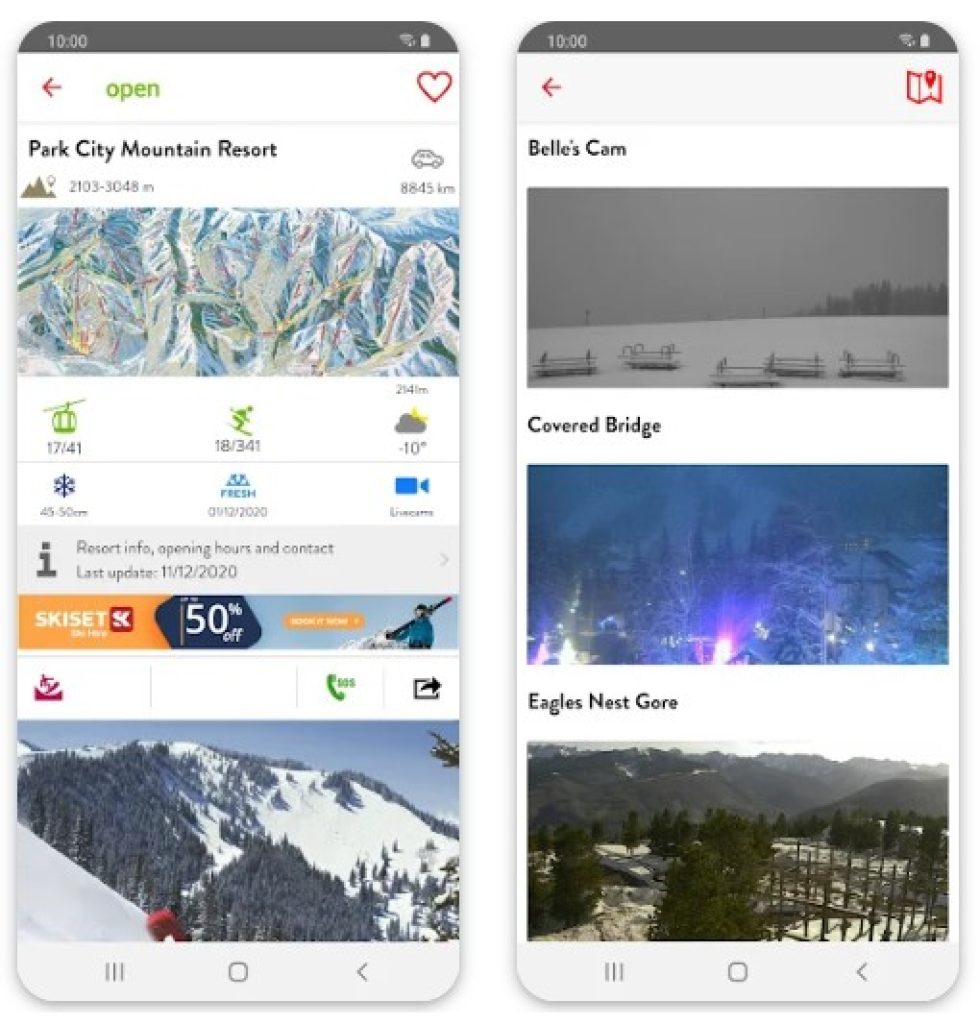This image is a split-screen comparison of two mobile phone displays showing information related to a ski resort. On the left side, the screen features a red arrow pointing left, accompanied by green text labeled "open" and a red heart symbol. Below this, in black text, it says "Park City Mountain Resort," followed by some detailed information, including mileage. A picturesque image of a mountainous region dominates the middle section of the screen, surrounded by three icons representing skiing, weather, and snow conditions, specifically noting "fresh" snow, along with a camera icon.

Beneath this image, a gray bar contains black text that provides "Resort info, opening hours, and contact" details, updated last on 11-12-2020. An advertisement banner for "Ski Set 50% off" follows below. At the bottom of this side, there's another image showcasing a snow-covered mountain with numerous trees.

On the right side of the comparison, the mobile screen displays three labeled photos. The top photo is from "Bells Cam," showing a snowy landscape. Below this, another photo labeled "Covered Bridge" displays more snow, lights, and trees. The last photo, "Eagles Nest Gore," highlights a mountainous terrain densely populated with trees.